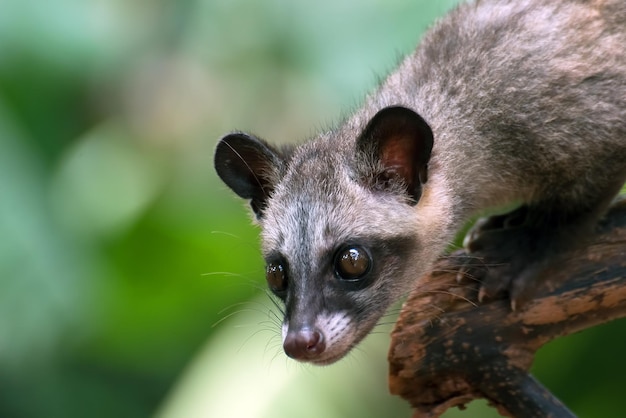This is a detailed close-up photo of a small, furry mammal, possibly a weasel, marmoset, or Civet, characterized by its striking features and vibrant setting. The animal, depicted from around the midsection up, has a mix of black, gray, and light brown fur, with noticeable dark ears trimmed with a hint of pink on the insides. Its large brown eyes and closed mouth give it a focused, observant expression. The animal is perched on a brown wooden branch, gripping it with visible black feet and sharp claws, clearly captured in an attentive pose. The background is a lush blur of predominantly green tones, likely tree leaves, suggesting a forested or wooded environment. The image is well-lit, indicating it was taken during daytime, and there are no text or numbers visible in the picture.